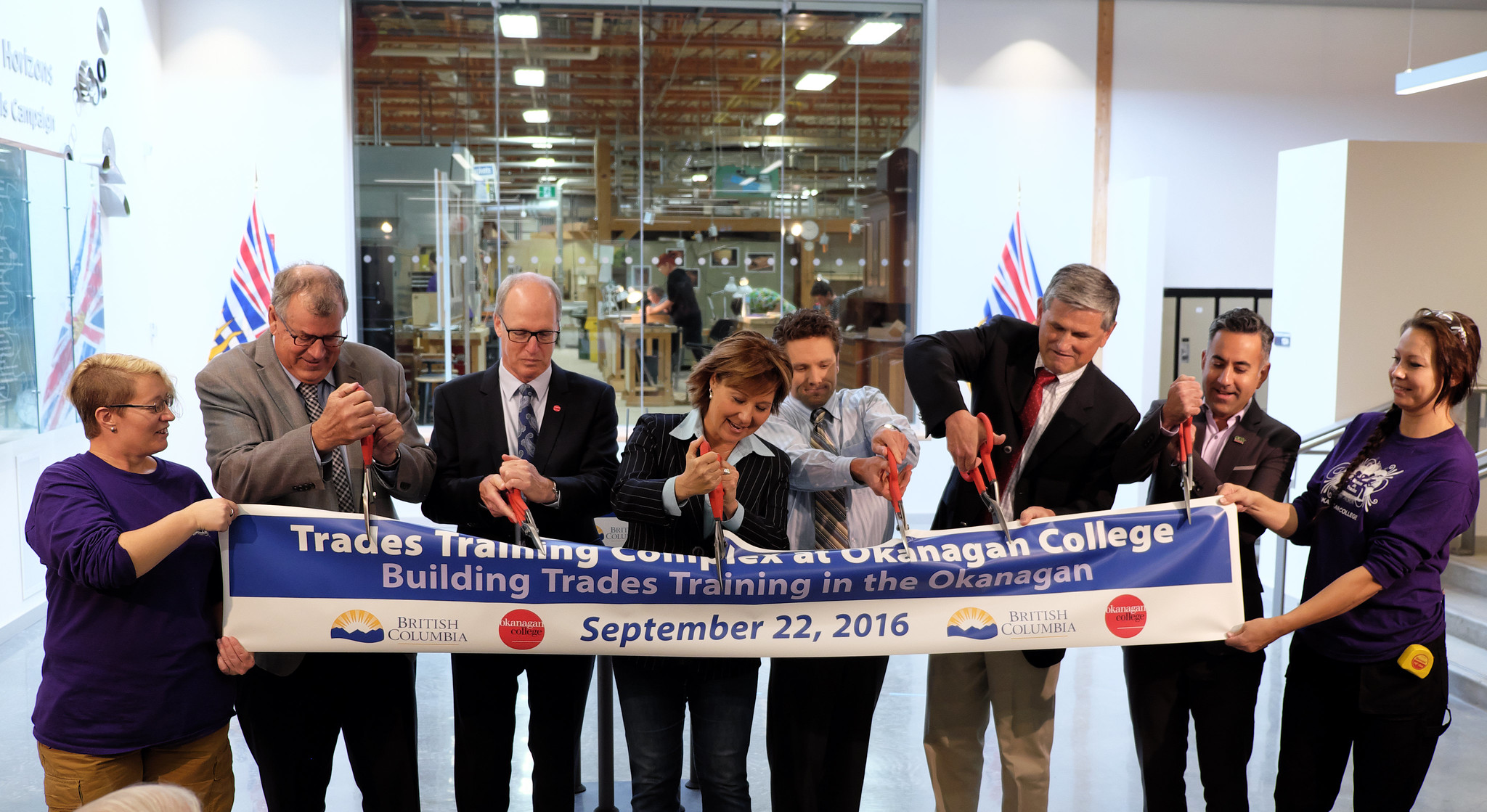This photograph captures a vibrant indoor ribbon-cutting ceremony for the Trades Training Complex at Okanagan College, which took place on September 22, 2016, in British Columbia. The center of the image features eight well-dressed individuals, all smiling and participating in the ceremonial cutting of a long blue and white banner. Each person holds a pair of scissors and the banner prominently displays the text: "Trades Training Complex at Okanagan College, Building Trades Training in the Okanagan, September 22, 2016, British Columbia." Flanking either end of the banner are two women, each lifting it up. The backdrop is brightly lit, showcasing expansive glass windows through which people can be seen working. Two prominent Canadian-British flags are visible behind the participants. The environment, likely an office or training facility, also features overhead lighting and a ceiling with notable brown accents. Colors in the scene include red, yellow, blue, white, beige, gray, black, and dark blue, creating a dynamic and festive atmosphere.